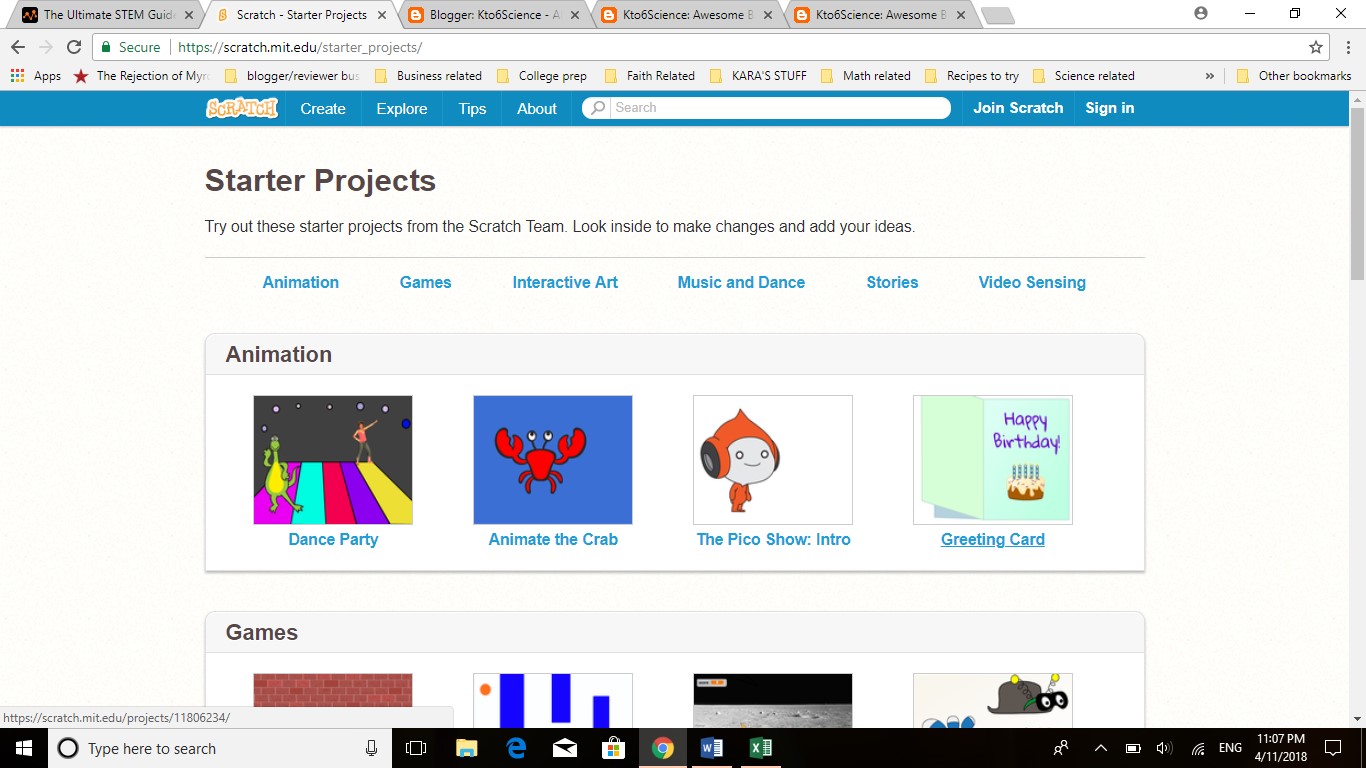The image appears to be a well-crafted mockup designed to resemble a screenshot of a monitor. It features a search result page from Bing displayed on what looks like a MacBook screen. The search query pertains to starter projects, specifically focusing on animations and games. Prominently featured are four results: "Dance Party," "Animate the Crab," "Pyco Show Intro," and a greeting card project. Each project is accompanied by a small, colorful illustration that adds a visual appeal to the page.

The background of the results page is primarily beige, with a contrasting blue band at the top that houses the search bar and Bing branding. The design is cluttered with text, offering options such as signing in to start a project, making it clear that the platform in question is Scratch, which specializes in beginner-friendly graphic design and coding activities. The vibrant illustrations and the organized layout make the mockup both informative and visually engaging, providing a comprehensive overview for anyone interested in diving into animation and graphic design using Scratch tools.